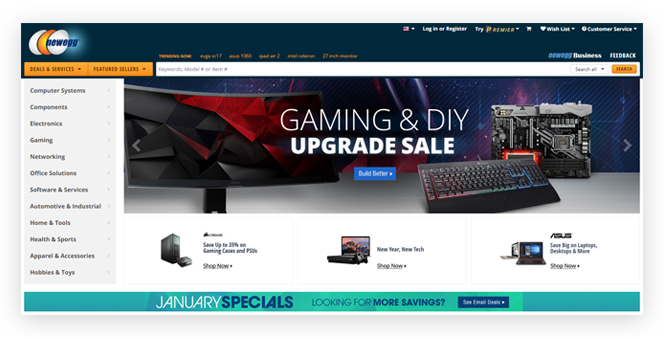A detailed and cleaned-up caption for the described image from the Newegg website could be:

"This is a cropped screenshot of the Newegg website's top section. The header features a black banner with the Newegg logo prominently displayed in the top left corner. On the top right, a drop-down box marked with the American flag indicates the English language setting. Adjacent to this, the options to 'Log in or Register' are written in small white letters. Further to the right are links for 'Wish List' and 'Customer Service,' followed by text indicating 'Newegg Honolulu' and a feedback icon. Below the black banner, there's an orange drop-down box labeled 'Sales and Service' next to a white drop-down box for 'Featured Sellers.' Extending across the banner is a long search bar; on its right end, there is a drop-down box defaulted to 'Select All' next to an orange rectangular search button.

On the left side of the main page body, there is a vertical gray sidebar listing various categories. To the right of this sidebar, a large promotional image dominates the page, announcing a 'Gaming and DIY Upgrade Sale' with a centered text overlay. Below this text, a blue button labeled 'Build' invites users to engage further. At the bottom of the screenshot, three thumbnails are displayed, each with product names and a 'Shop Now' hyperlink beneath them."